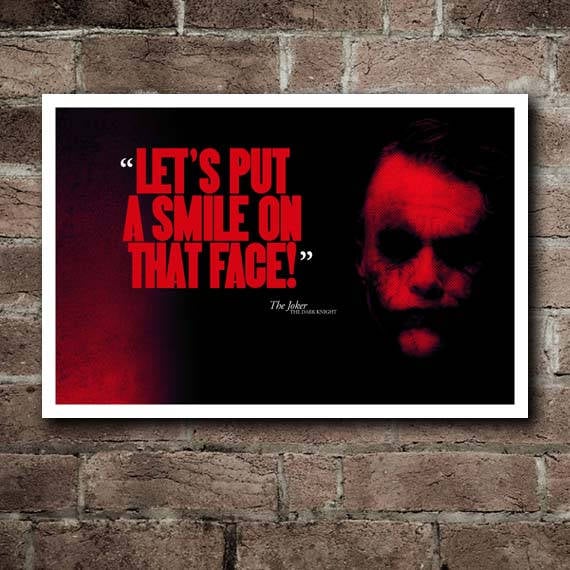This photograph captures a striking poster mounted on a rough-looking red brick wall. The poster features a prominent and eerie depiction of the Joker's face, characterized by exaggerated, messy makeup and shadowed, blackened eyes and mouth, all tinted in a vivid red. The unsettling image of the Joker is set against a solid black background, creating a stark contrast. Dominating the poster are large, bold red letters that spell out, “Let’s put a smile on that face,” enclosed in white quotation marks. Below this ominous quote, the words "the Joker" are printed in small white text, crediting the infamous character from "The Dark Knight." The entire poster is bordered by a clean white frame, which sharply delineates it from the rugged texture of the brick wall behind.